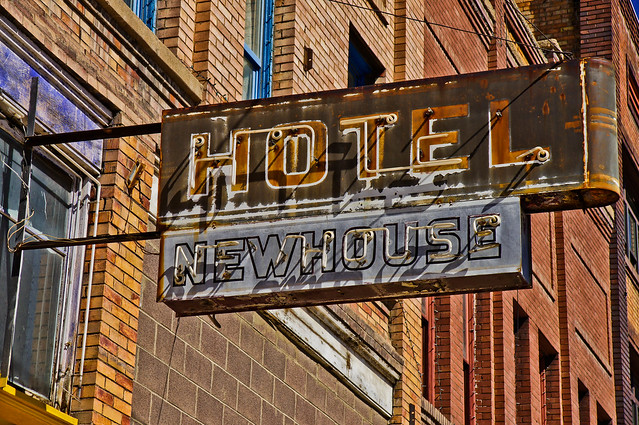The photograph captures a weathered neon sign mounted on a brick building’s facade, captured during the daytime with natural lighting. The square image focuses on the sign that juts out from a window of a multi-colored brick structure. The building itself features hues of red, gray, and light brown bricks, with additional yellow-tinted bricks visible to the left side. The scene includes no distinct background or border, only the adjoining sides of neighboring brick buildings, a few scattered windows, and no visible people.

The sign is distinctly aged and deteriorated, with visible rust and faded colors, suggesting it has not been maintained for quite some time. At the top part of the sign, which suffers extensive rust, the word “Hotel” is displayed in brown lettering, accompanied by neon tubing, much of which is broken or missing, making it unlikely the sign still functions. Below, a smaller portion of the sign, painted light blue, reads “New House.” This section also features neon tubes, though several appear damaged or absent, particularly affecting the letters “W” and parts of “E” and “L” in “Hotel.” The sign is affixed to the building by two metal rods and retains a nostalgic, albeit decayed, character emblematic of a bygone era.